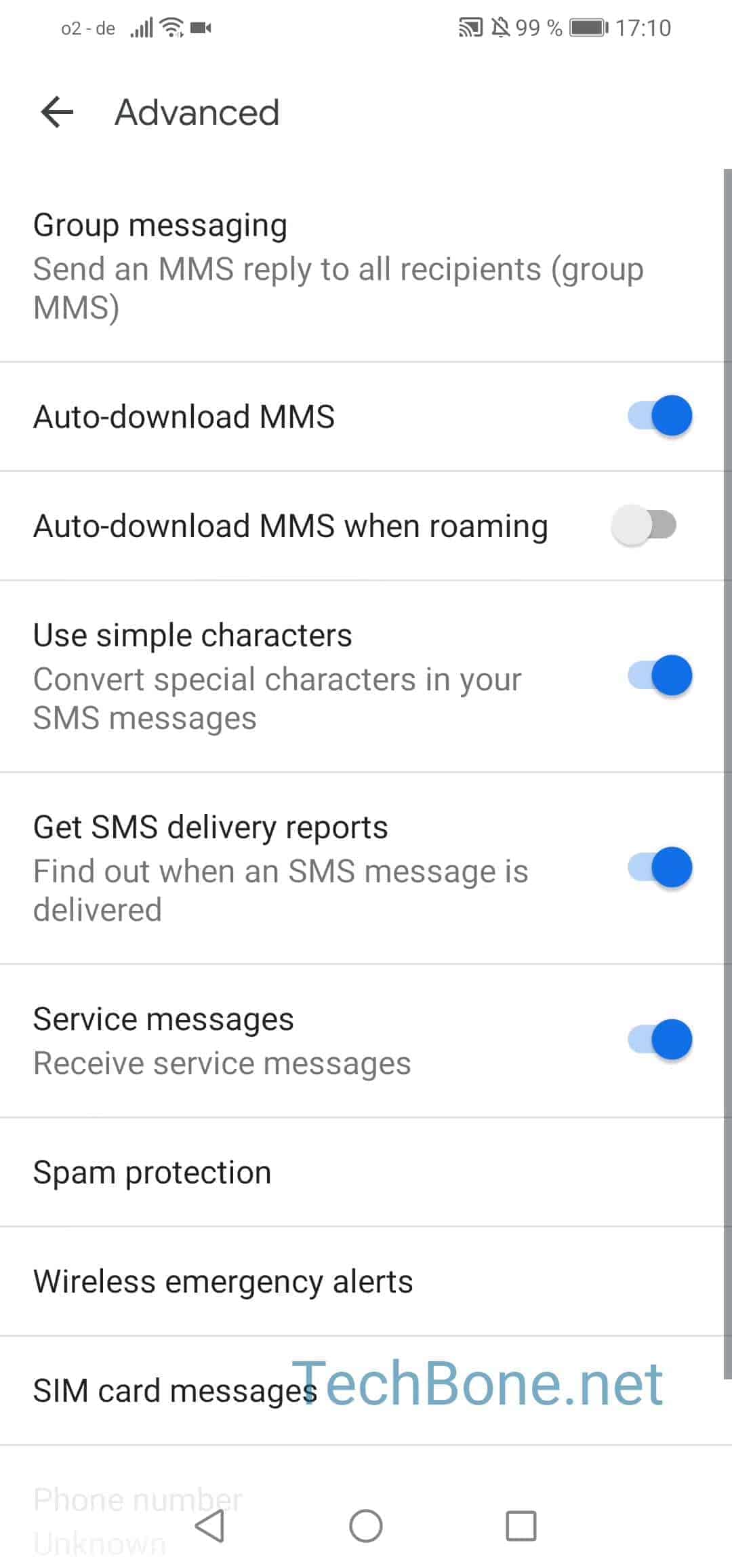Screenshot of a computer interface showing various messaging settings:
- At the top of the screenshot, there is a bar of computer icons.
- Below the icons, the word "Advanced" is displayed in black with a black arrow pointing to the left.
- Under "Advanced," the following settings are listed:
  1. Group Messaging: 
     - Description: "Send an MMS reply to all recipients." (Group MMS)
     - A thin gray line separates this from the next setting.
  2. Auto-download MMS: 
     - A toggle button for this option is turned on and appears blue.
  3. Auto-download MMS when roaming: 
     - A toggle button for this option is turned off.
  4. Use simple characters: 
     - Description: "Convert special characters in your SMS messages."
     - The toggle button is on.
  5. Get SMS delivery reports: 
     - Description: "Find out when an SMS message is delivered."
     - The toggle button is on.
  6. Service messages: 
     - Description: "Receive service messages."
     - The toggle button is on.
  7. Spam protection: 
     - There is no button displayed for this option.
  8. Wireless emergency alerts.
  9. SIM card messages:
     - Displayed in blue text: "TECHBONE."